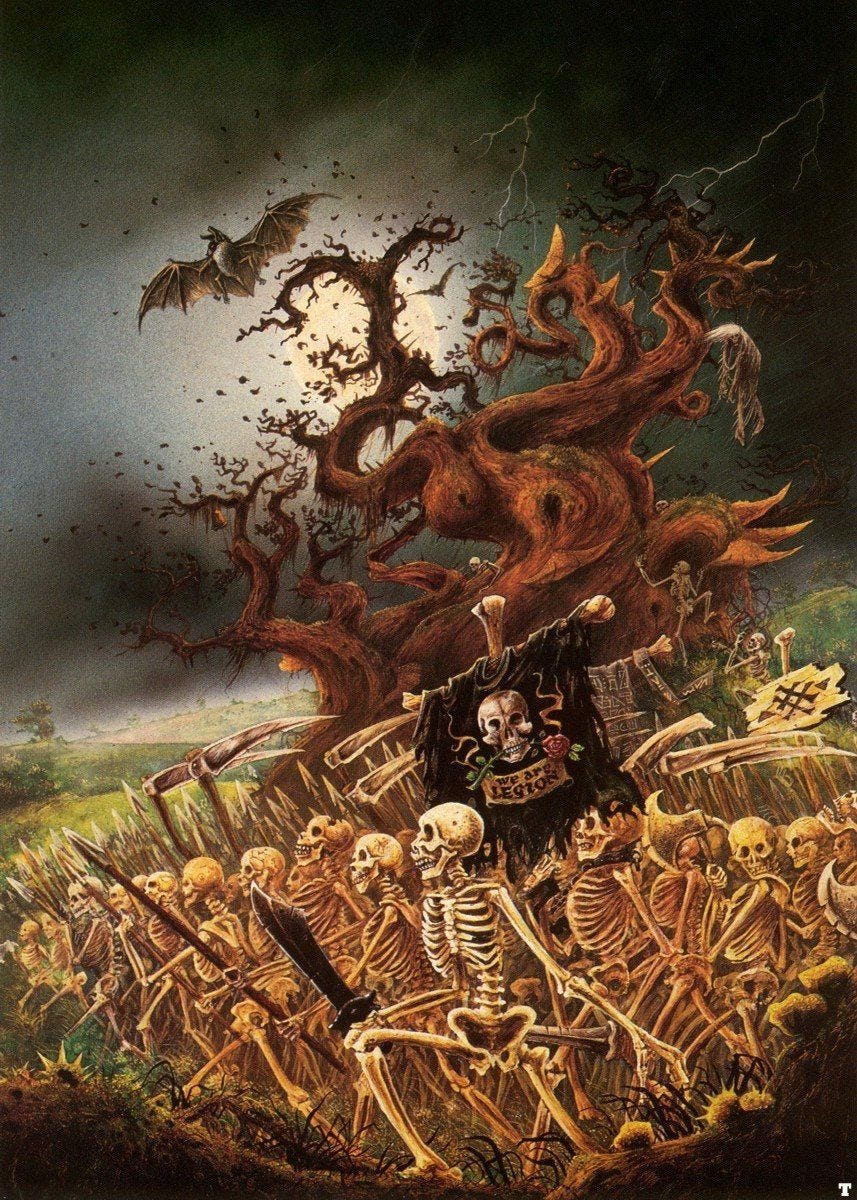In this eerie, fantasy-themed poster, the scene unfolds under a night sky cloaked in shades of black and gray, dominated by the haunting silhouette of a full moon. At the center stands a gnarled and twisted brown tree, devoid of leaves, its warped branches extending ominously into the dark. Emerging from the upper left corner of this sinister tree, a large bat with an impressive wingspan adds to the macabre atmosphere.

To the right of the tree, a flash of lightning pierces the gloom, casting brief illumination over a chilling sight. Surrounding the base of the tree, a fearsome army of 20 to 30 skeletons forms a chaotic but determined advance towards the left side of the image. The skeletal warriors are equipped with a variety of weapons: spears, knives, daggers, scythes, and axes, each one contributing to the menacing spectacle.

Amidst the ranks, a prominent skeleton brandishes a large black sword, leading the charge. Directly behind this commander, another skeletal figure hoists a black, shredded flag adorned with a skull clutching a rose between its teeth, flanked by golden snakes. Below the skull, a yellow banner bears the bold declaration, "We are Legion."

The bottom portion of the image transitions into green fields, creating a stark contrast to the dark and foreboding upper half. As the skeletal army rushes uphill, they are silhouetted against the eerie glow from the moon, their haunting forms casting long, jagged shadows across the desolate landscape.